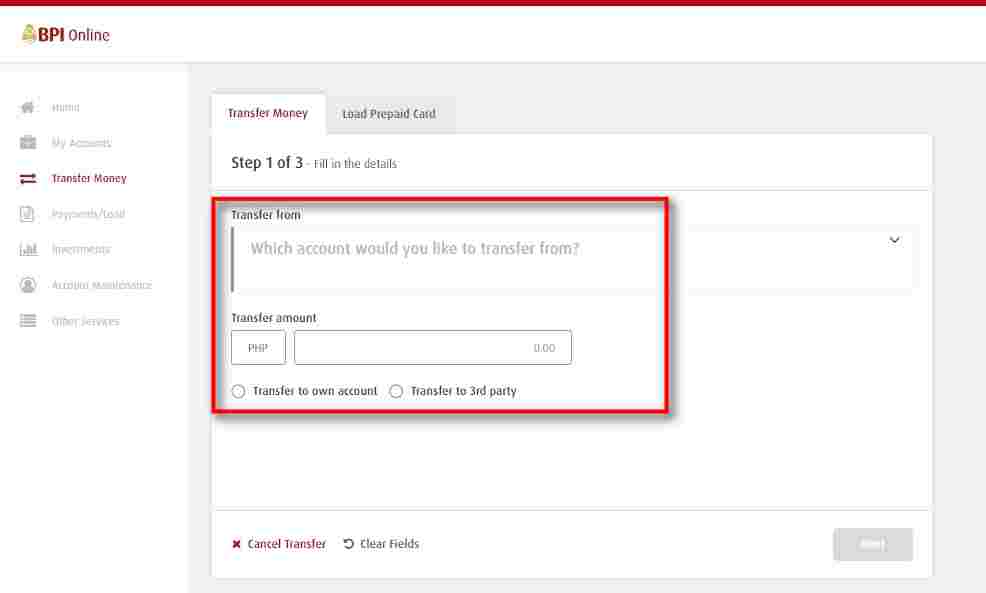A screenshot depicting an online banking interface with a white background. At the very top, a slim yet bold red bar spans horizontally, and just below it, 'BPI Online' is written next to a blurry logo, suggesting a possible association with the Bank of the Philippine Islands (BPI). The image quality obscures the logo. 

The screen appears to present the main dashboard or control panel of the online banking system. On the left side, there's a vertically arranged menu, each item accompanied by an icon. Though slightly blurry, the items seem to include "Home" or "My Account," with "Transfer Money" being the only clearly readable and highlighted item in red.

To the right, the interface transitions into a grey background section with white boxes. The top of this section reads "Transfer Money and Load Prepaid Card" in a folio layout, with "Transfer Money" selected. Below this, instructions are displayed: "Step 1 of 3: Fill in the details." A red-bordered box prompts the user to "Transfer From," asking which account to use for the transfer. There is also a field labeled "Transfer Amount, PHP," with the input box left blank.